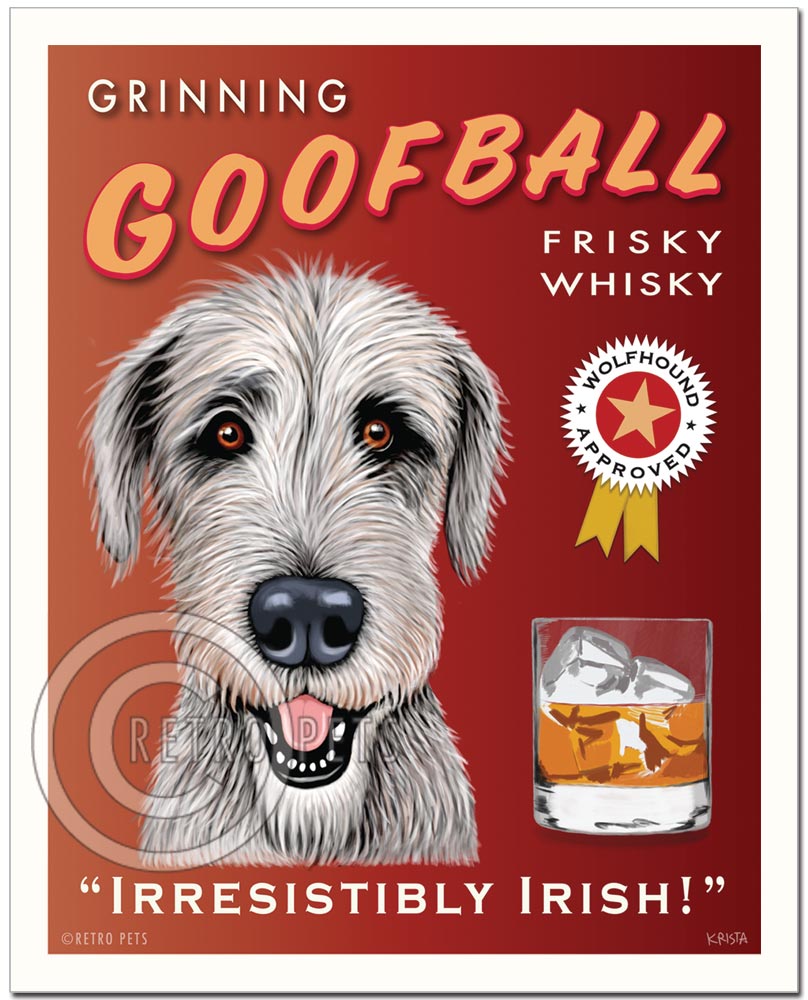The image is a portrait-oriented advertisement with a vintage, retro feel. The background transitions from dark orange to red, creating a fading effect. There is a darker cream trim around the edges, outlined in black. The centerpiece of the ad features a detailed drawing of a shaggy, silver-haired dog with a gray nose and brown eyes, staring directly at the viewer. Most likely a wolfhound, the dog's face dominates the left side of the image.

At the top left corner, the text "Grinning" appears in bold, white letters, followed by "Goofball" in orange with a red outline. On the right side, it reads "Frisky Whisky" in a matching style. A white jagged circle with a light yellow star in the middle and two gold ribbons states "Wolfhound Approved." 

In the bottom right corner, there is a detailed illustration of a whiskey glass with ice. At the very bottom, the tagline "Irresistibly Irish" is prominently displayed in large white letters. The ad also features a faded watermark at the bottom left, indicating the property of "Retro Pets."